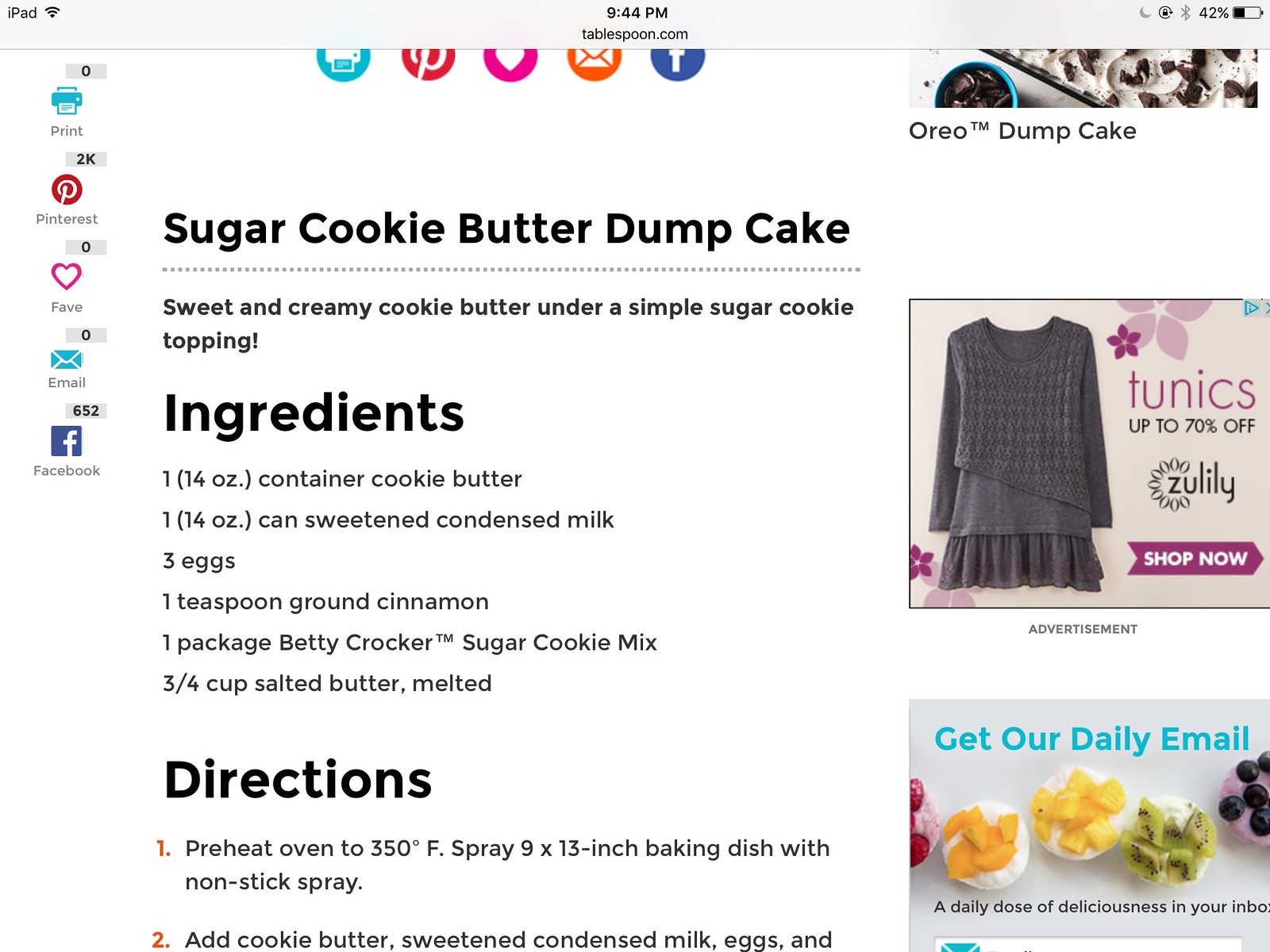This screenshot from Tablespoon.com, viewed on an iPad at 9:44 p.m., displays a partially visible web recipe for "Sugar Cookie Butter Dump Cake." The webpage features a clean, white background with several ads lining the right side, including promotions for Oreo Dump Cake, Zulily, and a daily email subscription. On the left side, the recipe text is in bold black and includes ingredients such as one 14-ounce container of cookie butter, a 14-ounce can of sweetened condensed milk, three eggs, a teaspoon of ground cinnamon, and a package of Betty Crocker sugar cookie mix, followed by ¾ cup melted salted butter. The directions begin with preheating the oven to 350°F and spraying a 9x13 inch baking dish with nonstick spray before being cut off. Along either the extreme left or right edges, there are icons for printing, Pinterest, Favoriting, Email, and Facebook, facilitating easy sharing and interaction with the content.